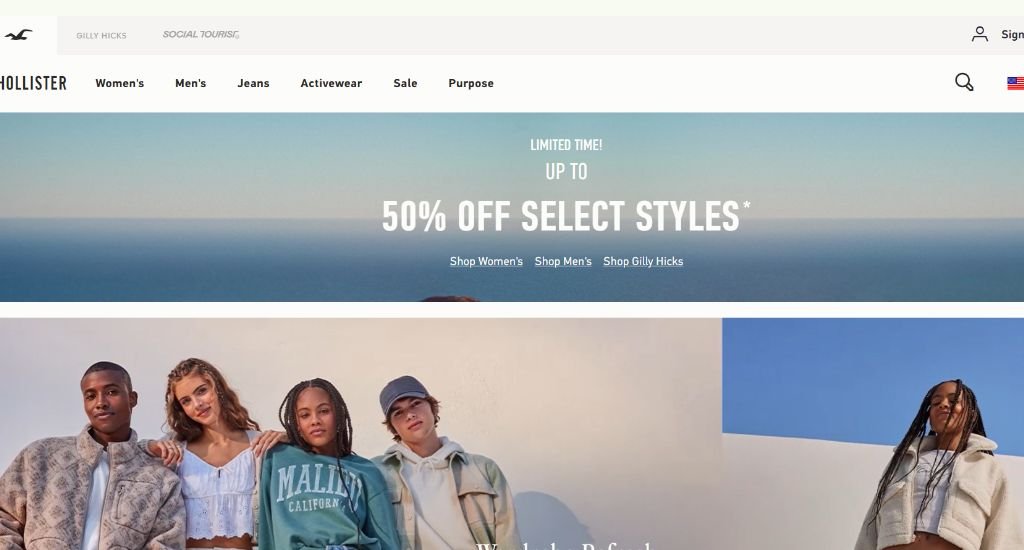The webpage features a navigation bar at the top with several tabs. The first tab displays an icon of a black bird flying to the left. Adjacent tabs include "Ghillie Hicks" and "Social Tourist." In the top right corner, there is a "Sign In" button. Below the main header, additional tabs are listed: "Hollista," "Women's," "Men's," "Jeans," "Activewear," "Sale," and "Portals." To the right of these tabs, there is a search icon accompanied by a USA flag featuring blue, red, and white colors.

Beneath these navigation tabs, a promotional text is prominently displayed against a background that features a serene blue sea and a slightly blue sky. The text is tall and reads: "Limited Time Up to 50% Off Select Styles. Shop Women's, Shop Men's, Shop Ghillie Hicks."

The bottom section of the webpage showcases another advertisement. On the left side of this ad, there are two males and two females wearing clothing from the store. The background here is brown. On the bottom right, another woman is pictured wearing a fluffy cream-white jersey over a white t-shirt, against a brown background. Above her head, there is a section of blue background.